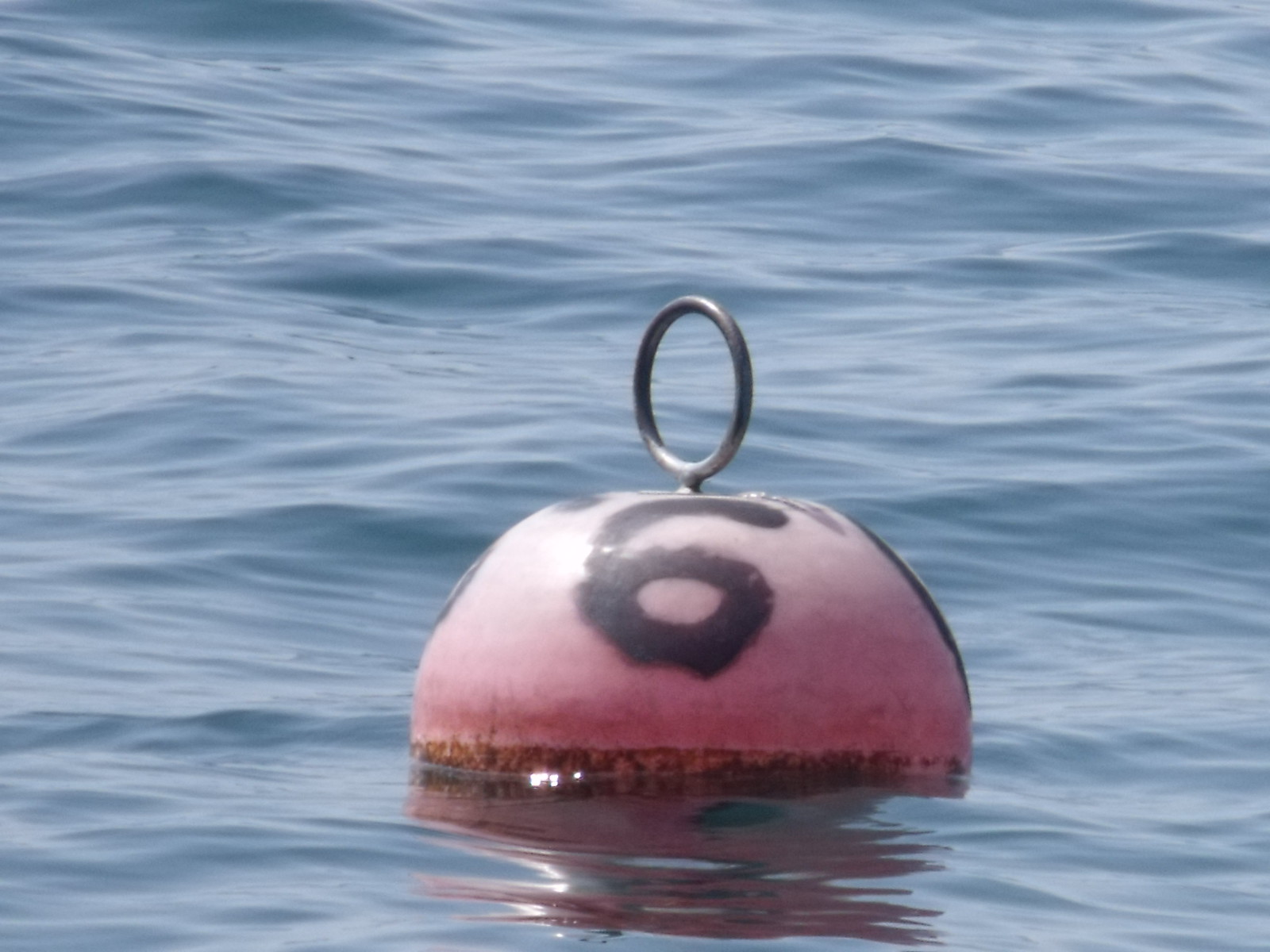This photograph captures a close-up view of a buoy floating in a body of water, likely the ocean, as suggested by the calm yet rippling waves surrounding it. The water, predominantly light blue with darker blue accents where it ripples, occupies the entire frame, reflecting sunlight and creating a bright, serene ambiance. The focal point of the image is a round buoy, its upper portion a reddish-pink color prominently marked by a free-handed, thick black number six, spray-painted in the center. The painted six has uneven edges, indicating it was added manually rather than manufactured. The buoy exhibits a distinct horizontal waterline, below which its surface shows signs of weathering with orange rust, likely from prolonged exposure to saltwater. At the top of the buoy, a metal hoop, possibly stainless steel, is attached, appearing slightly smaller than the buoy's diameter and reflecting the sunlight. The hoop is presumably welded on for durability. The overall image conveys a sense of isolation and tranquility, with the buoy steadfastly floating amidst the gently undulating sea.